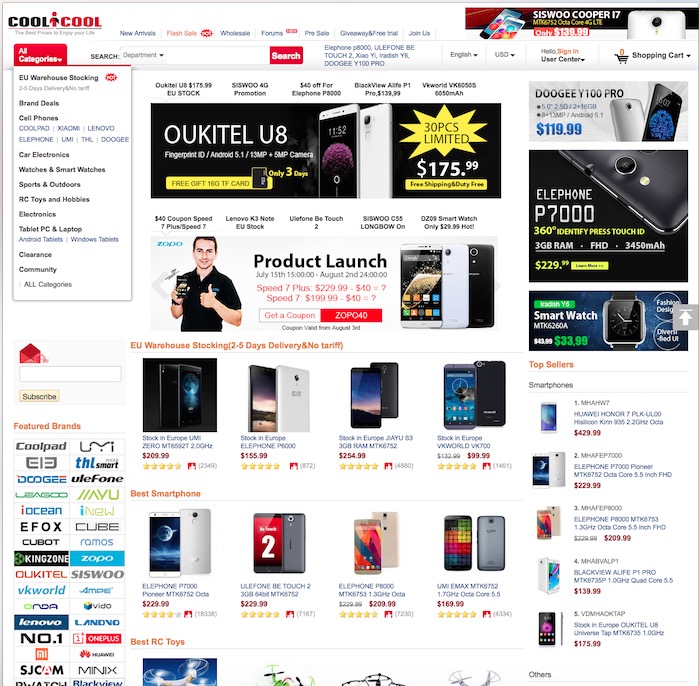This is a detailed screenshot of a bustling e-commerce website advertisement page for Cool Cool, featuring a sleek white background. At the upper left-hand corner, the company name, "Cool Cool," is prominently displayed. Below this sits an "All Categories" drop-down menu, accompanied by a search button and a subscribe button. In the lower-left corner, logos and colors of featured brands are showcased, adding a splash of diversity to the page.

The main content area is dotted with various electronic items, predominantly cell phones, each presented with clear photographs, prices in red text, and star ratings. The right-hand vertical column features three distinct advertisements. Among these is a section at the bottom labeled "Top Sellers," highlighting five smartphones complete with their respective prices.

Adjacent to the search bar, in the upper-right corner, are additional drop-down menus for language and currency options, alongside sections for signing in and accessing the shopping cart. The page's upper center displays two or three advertisements, including one for "OUKITEL U8" and another promotional banner titled "Product Launch," featuring an image of a man giving a thumbs up.

Overall, the page exudes a busy and vibrant atmosphere, designed to capture the attention of potential customers through a strategic mix of product placements and advertisements.